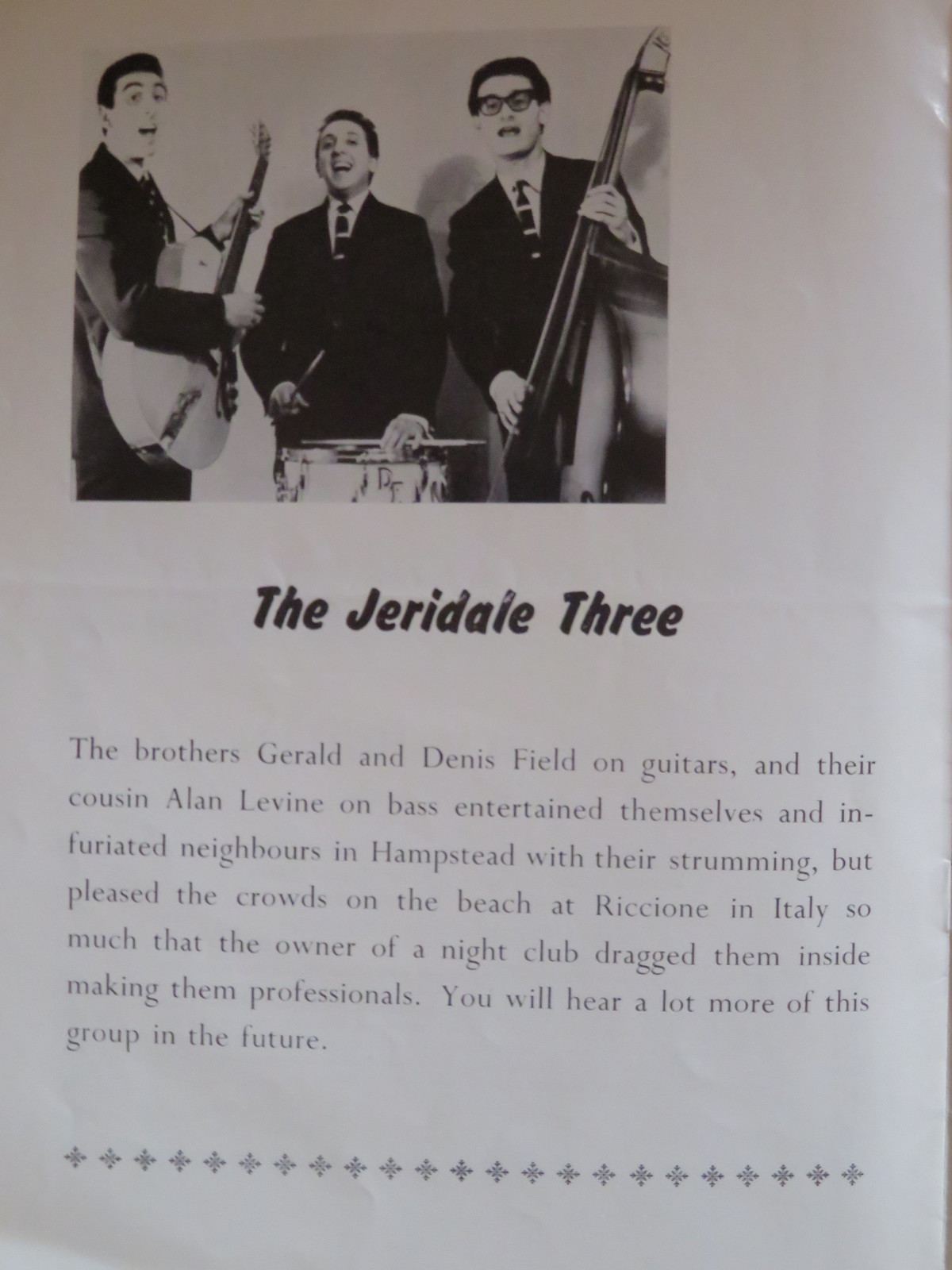The informational flyer features a vertical, white rectangular background with a black-and-white photo prominently displayed just left of center. The photo captures three Caucasian men wearing identical black suits with black and white striped ties. On the left, one man is playing a guitar and appears to be singing with his mouth open. The central figure is positioned with a drum—either a snare or bass drum—in front of him, also singing. On the right, another man is playing a cello and singing along.

Below the photograph, in bold black font, the text reads "The Gerardale Three." The accompanying text introduces the band members: brothers Gerard and Dennis Field on guitars, and their cousin Alan Levine on bass. The narrative humorously details how their musical endeavors in Hampstead brought pleasure to themselves but did not sit well with their neighbors. However, their performances on the beach at Riccione in Italy were so warmly received that a nightclub owner invited them to perform professionally. The flyer optimistically concludes that we will likely hear more from this talented group in the future.

The bottom of the flyer is adorned with a diamond-shaped border running horizontally from left to right, providing a polished finish to the design. The overall effect is a stylish, monochromatic poster designed to introduce and promote the upcoming band, The Gerardale Three.